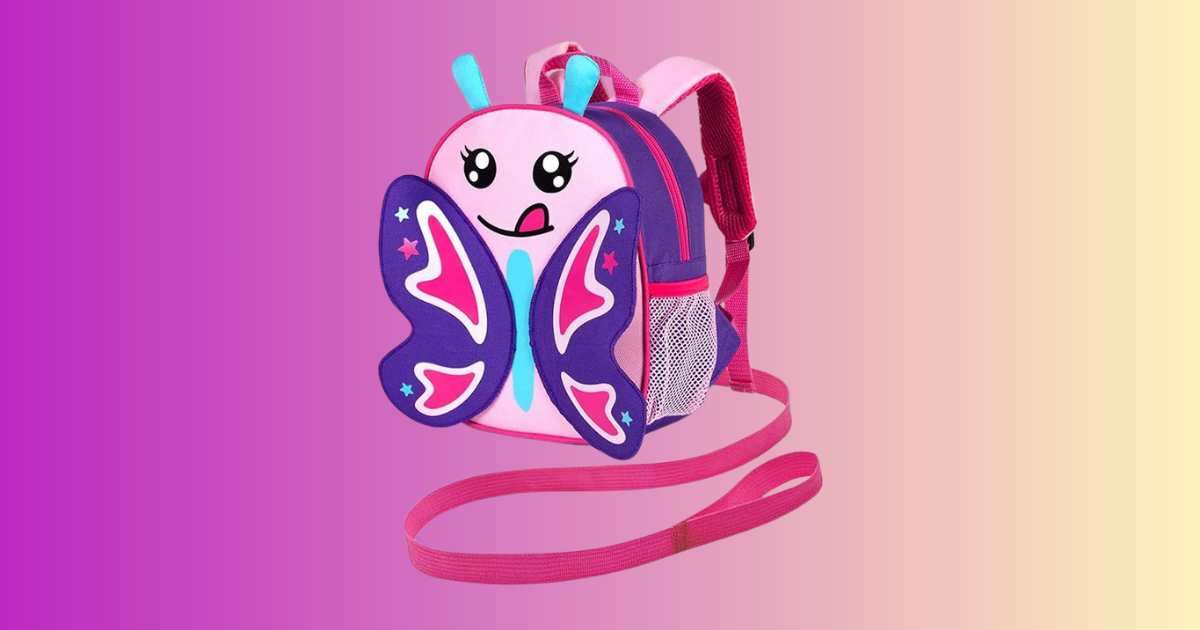The image depicts a child’s backpack designed as a playful butterfly. The backpack itself is predominantly pink with various shades ranging from light to dark. Its front side is adorned with animated, black-and-white eyes and a cheerful smile featuring a pink tongue. The butterfly theme is emphasized by decorative purple and pink wings, which are detailed with little stars and a variety of pink shades. The butterfly’s body, positioned between the wings, is a light powder aqua blue. On top of the backpack, two powder blue ears function as the butterfly’s antennas. It also includes functional elements such as a mesh drink holder and adjustable pink straps, making it both practical and adorable for young children. The background of the image features a gradient transitioning from yellow to orange to purple, adding a vibrant and whimsical touch.